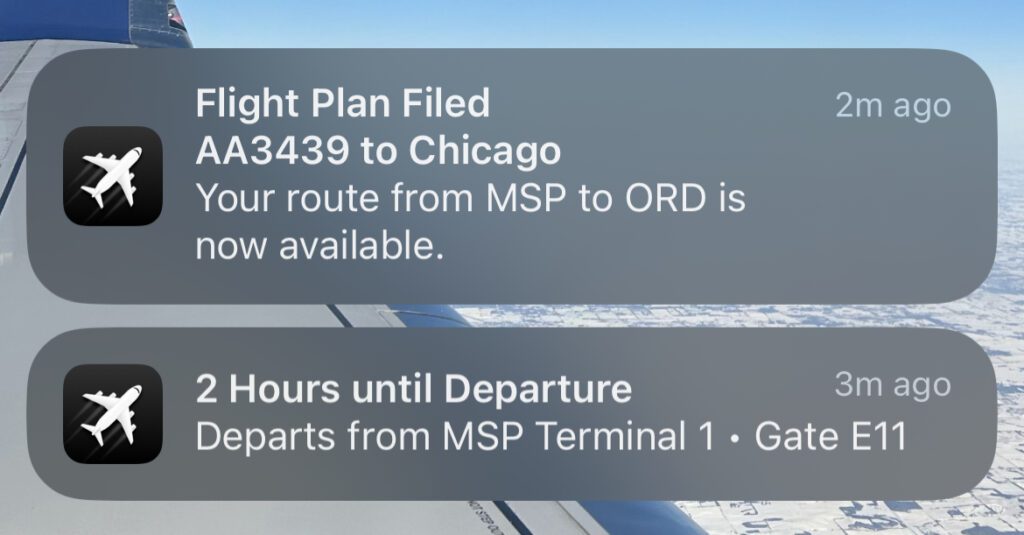Detailed Caption:

The image is a screenshot depicting a flight management interface, where users can either register for a flight or receive flight reminders. The primary focus of the image is a gray rectangular text box with rounded corners containing concise flight updates. On the far left side of the text box, there's a white airplane icon displayed within a black rounded square. The first message indicates that it arrived two minutes ago and states: "Flight plan filed, AA3439 to Chicago. Your route from MSP to ORD is now available."

Below this, there is a similar gray text box with the same airplane icon. It contains a message received three minutes ago, providing a countdown: "Two hours until departure. Departs from MSP Terminal 1, gate E11."

The background of the screenshot features a view from an airplane window, capturing the aircraft's wing and extending over a snowy cityscape, which is complemented by a broad sky in the distance. The snow-covered land below adds a crisp, wintry atmosphere to the scene.